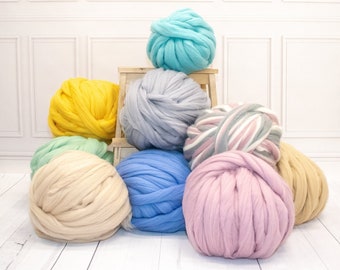In the image, nine balls of thick, ropey strips, resembling yarn, are arranged in a neatly wrapped cluster in front of a lightly-colored wooden step stool. The floor underneath them is made of white wooden tiles, and a pristine white wall serves as the backdrop. The balls of cloth are varied in color, creating a vibrant display. The ball closest to the viewer is light pink, positioned beside a mix of white, pink, and black. To their right, another ball stands out in bright canary yellow. At the bottom center lies a blue ball, on top of which rests a gray one, with a light blue ball also visible. To the left of the blue and gray balls is a green one, and in front of the green ball lies a tan-colored one. The arrangement is orderly and the setting appears clean and well-lit.